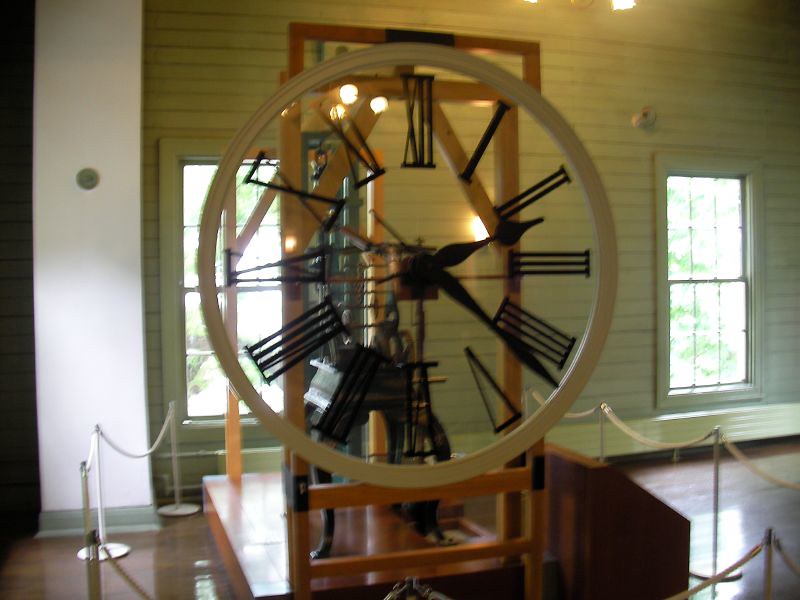A slightly out-of-focus photograph captures the imposing presence of a large clock face displayed in a museum-like setting. The clock, mounted on a stand, dominates the foreground, its white face adorned with Roman numerals and Gothic-inspired large hands, indicating the time as 2:21. The intricate wooden frame holding the clock is clearly visible, showcasing craftsmanship against a backdrop of a room characterized by varnished dark wood floors and green skirting. The room features a white wall at the front, contrasting with the pale green horizontal wooden cladding behind the clock, suggesting windows or another form of open space. Surrounding the clock and its stand are cordons with ropes, ensuring the exhibit remains undisturbed. This grand timepiece is elevated on a raised wooden platform, further emphasizing its prominence in the exhibit.